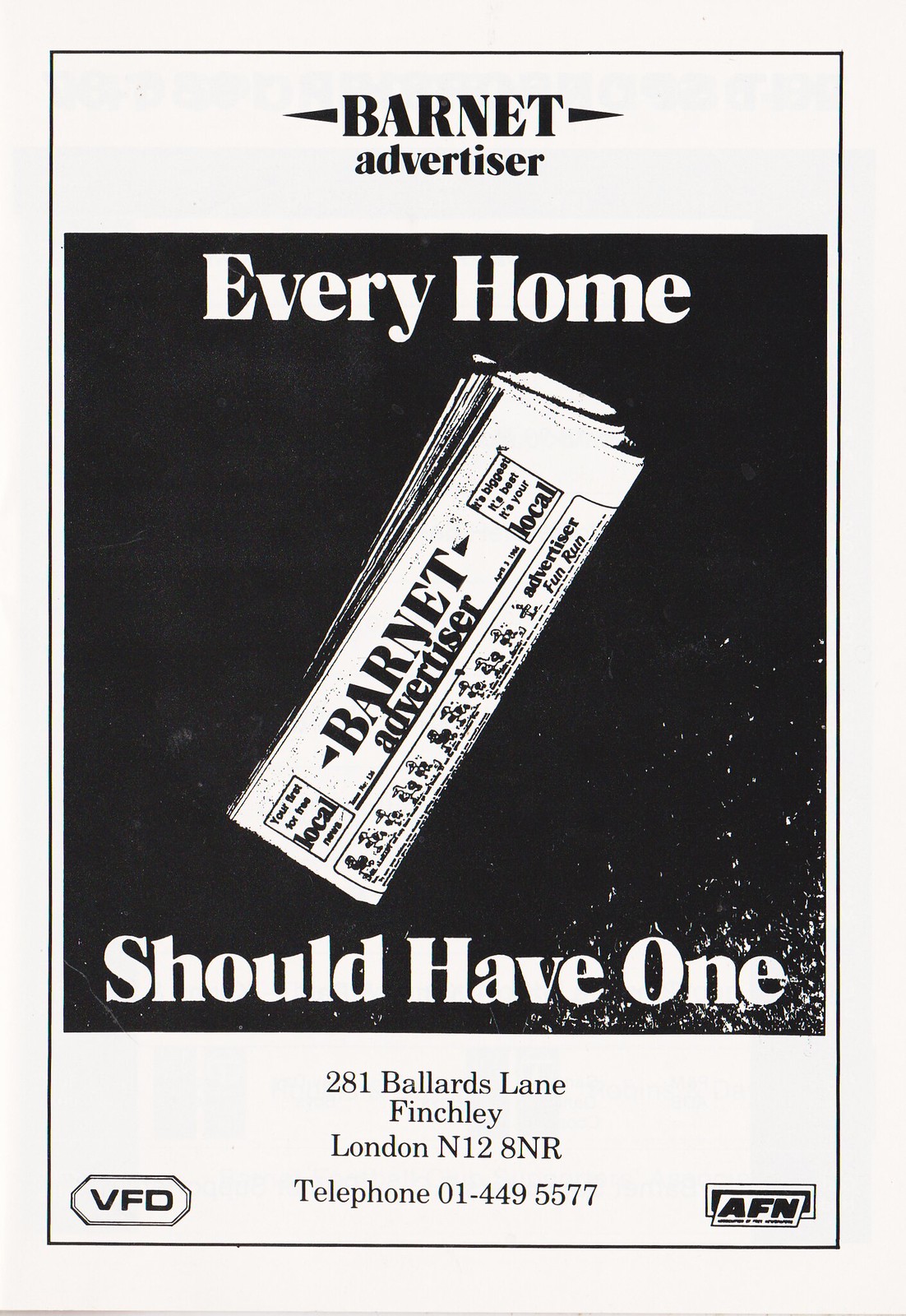The image is a black-and-white advertisement for the Barnett Advertiser. At the very top, the title "Barnett Advertiser" is written in black, flanked by arrows pointing left and right. The background of the image transitions to black in the center, covering about 75% of the layout. In the center, the bold white text reads "Every Home Should Have One." Diagonally positioned from approximately 7 o'clock to 1:30, there is a folded newspaper displaying "Barnett Advertiser" and additional but unreadable text. At the bottom of the black area, "should have one" is written in white text.

Returning to a white background at the bottom, the address "281 Ballard's Lane, Finchley, London, N12 8NR" is listed in black text, followed by the telephone number "01-449-5577." In the bottom left corner, a black hexagon-like logo with "VFD" is noted, while in the bottom right corner, a black logo with "AFN" is present. The entire advertisement maintains a simple black-and-white color scheme.